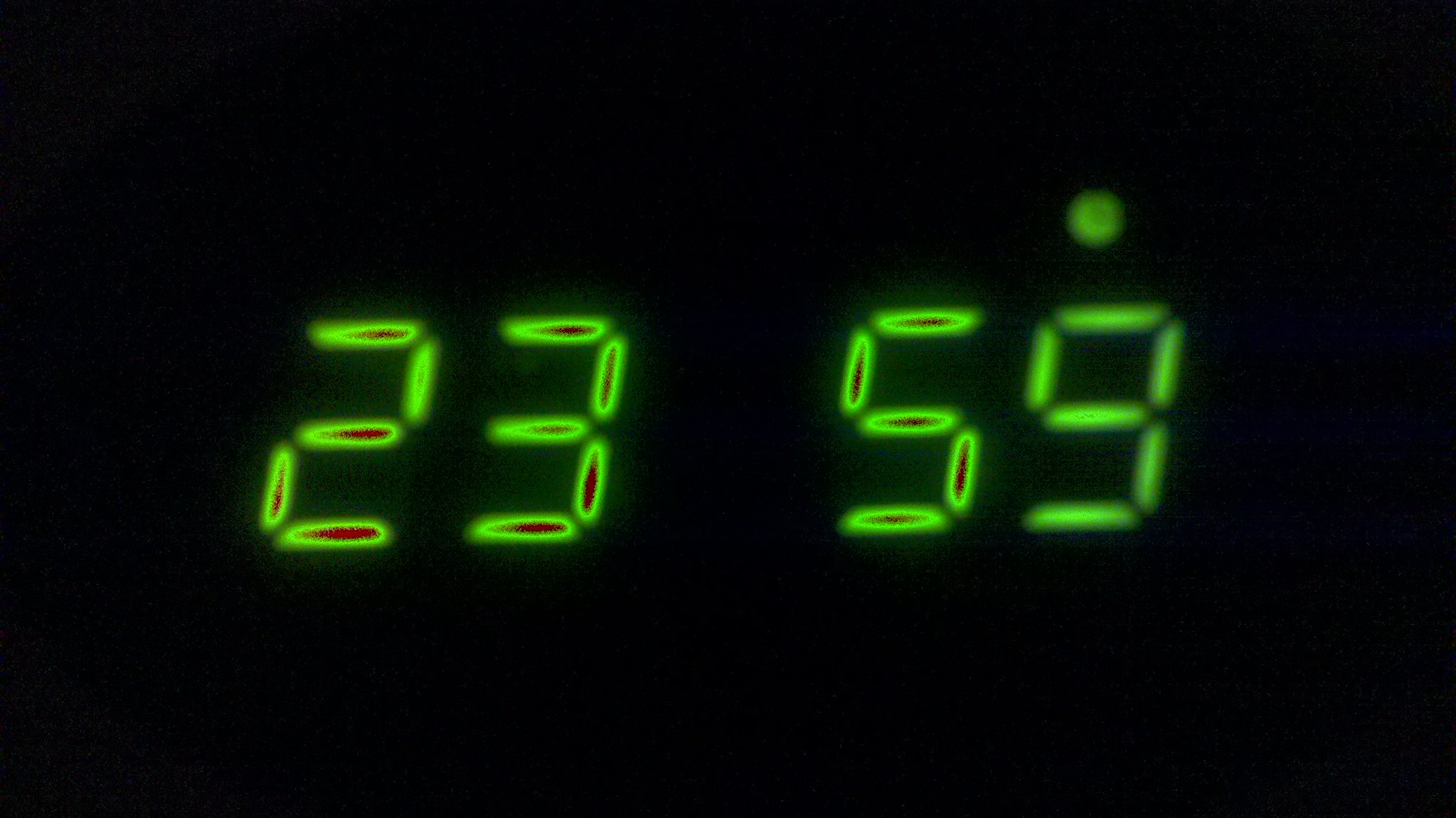The photograph is a color close-up of a vintage 80s-style LED clock displaying the time "23:59" against a completely black background. The segmented numbers “23” and “59” are positioned centrally, with a noticeable green dot above the “9.” The numbers exhibit a neon green glow, characteristic of old digital clocks. Interestingly, the digits “2,” “3,” and “5” have a reddish tint in the center of their segments, while the “9” and green dot do not exhibit this peculiar coloration. The image may have undergone digital alteration, but no text or markings confirm this speculation. The clock’s digits and dot appear slightly fuzzy rather than crisp, especially around the “9.” This detailed and focused shot captures the unique aesthetic of an illuminated LED display in total darkness.